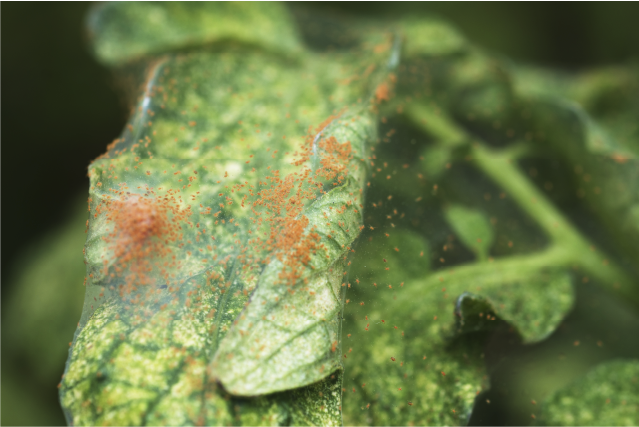This detailed close-up photograph features a green, veined leaf, possibly from a tomato or potato plant, that exhibits signs of distress. The leaf, which appears to be partially rolled up at the edges, has both areas of focus and blur: the left side is sharper and highlights the intricate vein patterns, while the right side is blurred. A notable feature of this image is the presence of numerous small, orangey-red specks scattered primarily on the left side of the leaf. These specks may be indicative of an agricultural pest or disease, such as mites or fungal spores. These orange-red particles seem to rest on or near a cloudy material, possibly resembling a spider's web, adding to the texture around the leaf. The overall health of the leaf appears compromised, as suggested by the chlorotic (bleached and yellowing) patches amidst the green foliage, pointing to possible insect damage or infection. The scene is framed centrally with no text, emphasizing the leaf's unhealthy state and the suspicious red specks as the primary subjects of this photograph.